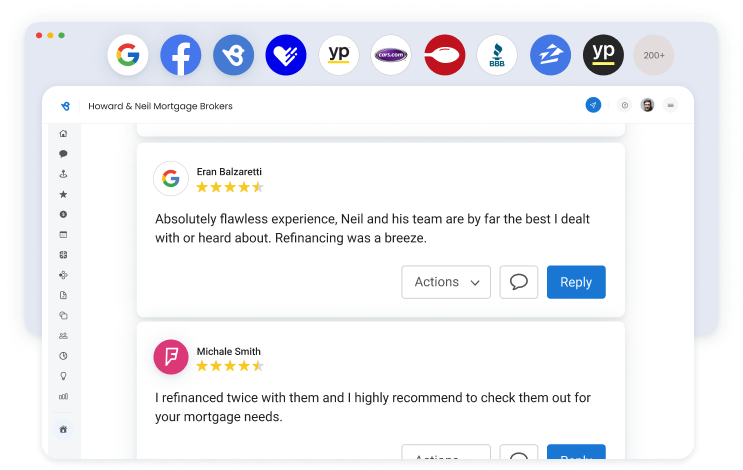**Descriptive Caption:**
The screenshot features a user interface with a distinctive gray and bluish-gray circular background, resembling a sideways phone screen. At the top left corner, there are three iconic buttons: red (close), yellow (minimize), and green (maximize), typical of a window's control panel. Below these controls, an array of icons is displayed, including recognizable logos for Google, Facebook, a fragmented heart, YP (Yellow Pages), a blue icon, potentially linked to a major brand, and more. Among these, there's an icon resembling Betty Crocker's spoon, one featuring a torch, and another black icon with yellow text reading "YP," followed by "200+" indicating additional items.

The main content is divided into two sections. The upper section prominently displays the header "Howard and Neal Mortgage Brokers" with clickable buttons next to it. Underneath, there are multiple icons aligned vertically, estimated to be at least 12. The lower section contains highlighted testimonials. One review is from a Google user, almost five-star rated, praising Neal and his team's exceptional refinancing service. Another review from Michelle Smith, also nearly five-star, speaks highly of her twice-refinanced mortgage experience with the brokers, recommending them for mortgage needs. These testimonials appear as clickable snippets for detailed viewing.